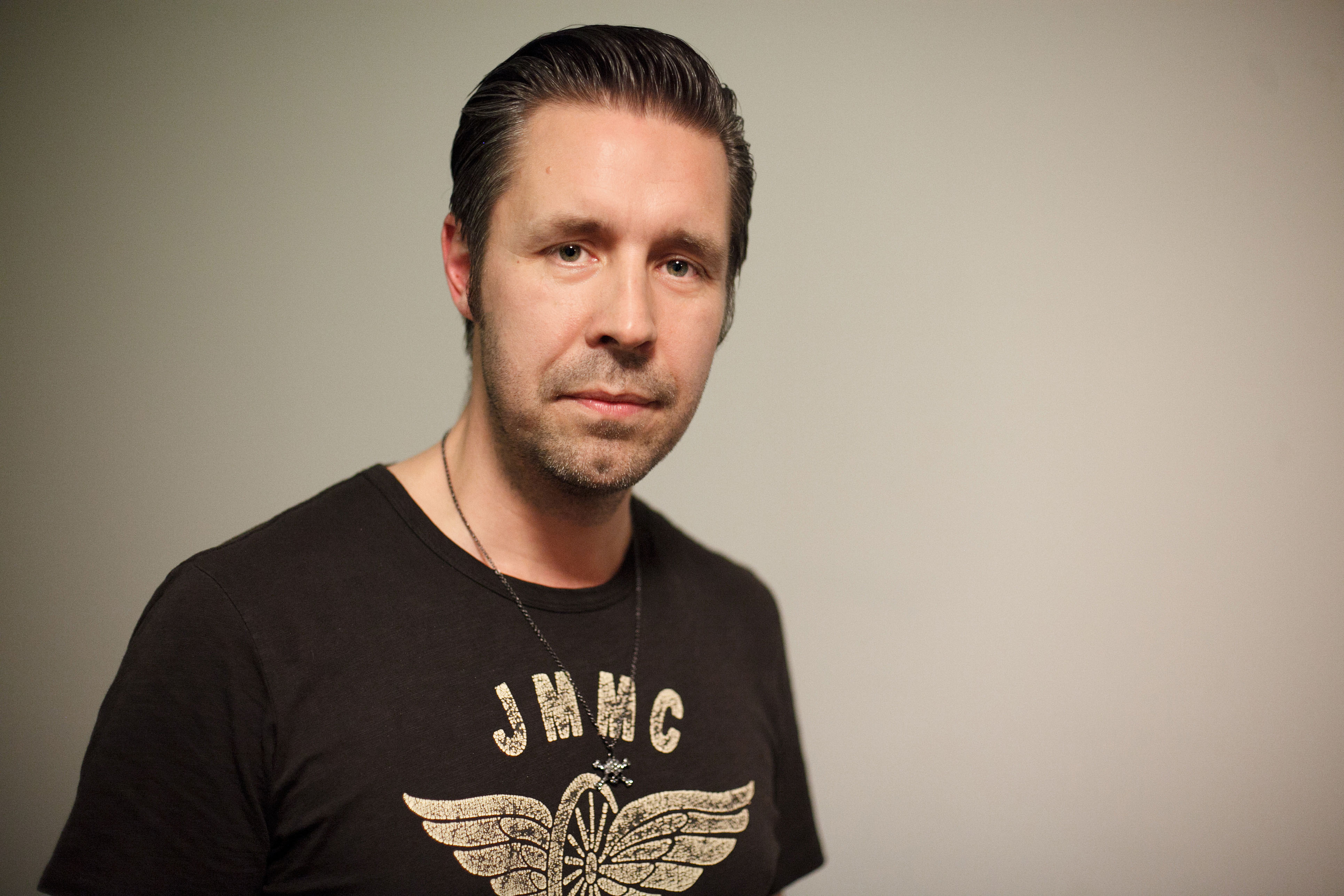In this digital photograph, a middle-aged man is positioned to the left of the frame, occupying the left half of a landscape layout against a plain gray background. The right half of the image is empty, emphasizing the man's presence. He gazes directly into the camera with a stern, perhaps slightly sad expression. The man appears to be in his late 30s or early 40s, with short brown hair slicked back, possibly using gel which gives it an oily sheen. His light brown eyes are surrounded by stubble peppered with a few specks of gray in the beard and mustache area.

He is wearing a black t-shirt adorned with a worn-out white print that reads "JMMC" at the chest, beneath which is an illustration of an old wagon wheel with wings. Additionally, the man wears a necklace made of thin black fabric and a small silver pendant, its specific shape difficult to discern but possibly resembling a skeleton crossbones. The simple yet detailed composition draws attention to the man's contemplative demeanor and subtle details in his appearance and attire.